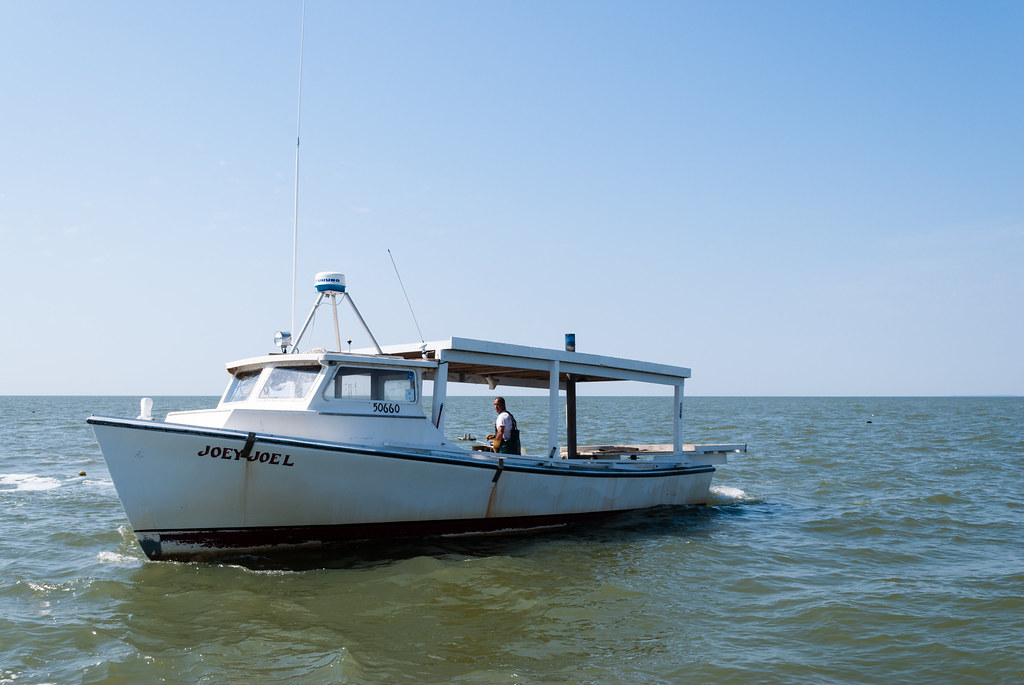The photograph captures the serene scene of an old, medium-sized fishing boat named "JOEY JOEL" drifting on a calm, moss-green ocean. The vessel, prominently white with sporadic rust spots and dark blue trim along the upper edge, features a wooden canopy at its stern. Inside the boat, a single man dressed in a white t-shirt and dark overalls stands near the center, looking back over his shoulder towards the camera. On the starboard side, he is positioned close to a fishing pole. Near the bow, the boat bears the registration number "50660" and displays its name "JOEY JOEL" in capitalized black font. Extending from the roof area above the captain's position is a long antenna that reaches almost out of the image’s frame. Additionally, a three-legged tripod with a blue and white round case at its summit, and a spotlight at the front of the covered area, are also visible. The backdrop features a vast, clear blue sky that transitions to a lighter shade of gray near the horizon, completing the tranquil maritime tableau.